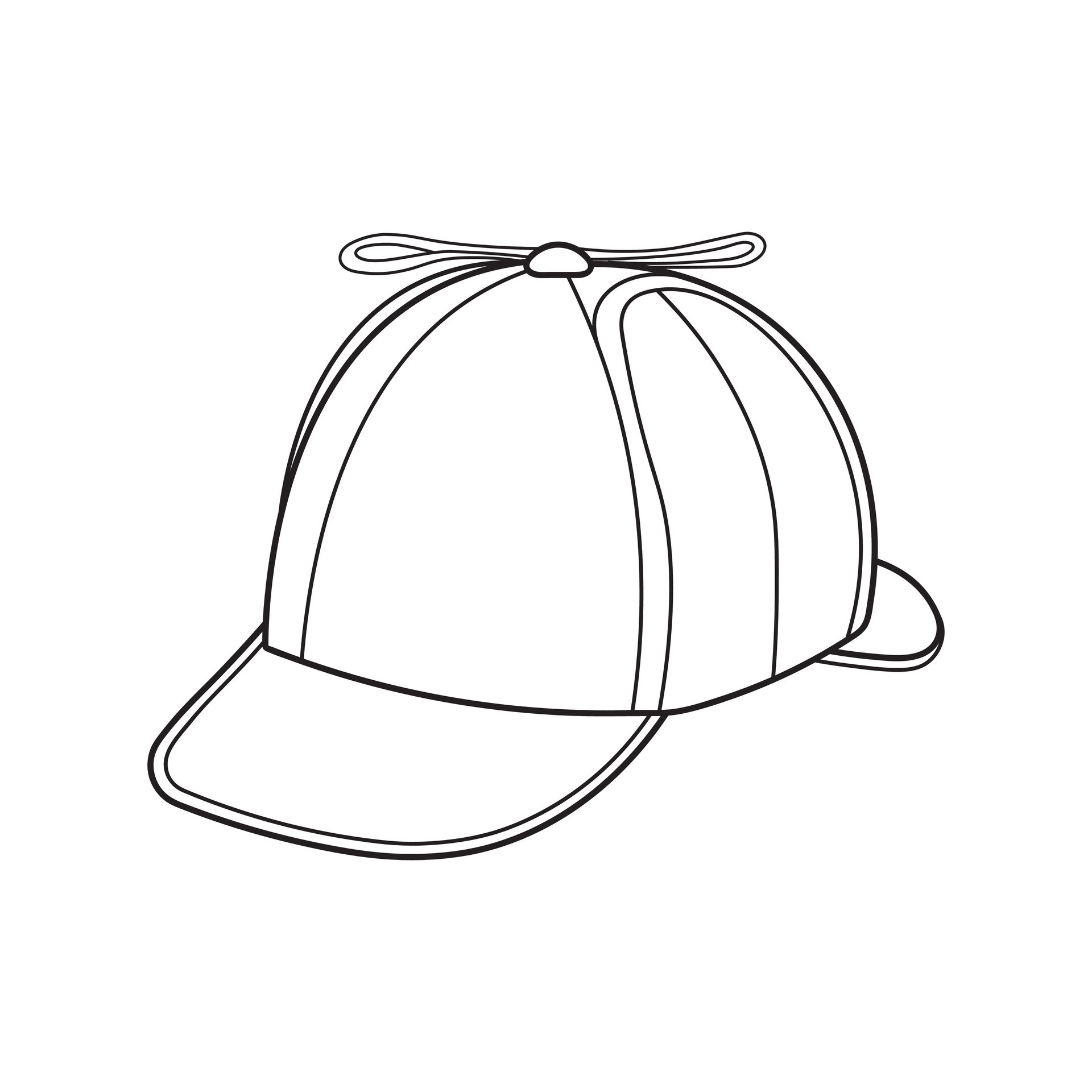This is a detailed black and white illustration of a whimsical hat, reminiscent of a propeller beanie, set against a stark white background. The hat is centrally positioned in the image, with the base of the dome-like top centered, and the front bill extending towards the bottom left. Another bill is partially visible behind it, positioned slightly to the right and overlapping the base. At the top center of the hat, there's a small circular button from which a propeller extends, with blades sticking out to the left and right. The drawing style is simple and unadorned, featuring minimalistic, clean, and unshaded lines, resembling artwork from a coloring book where the main purpose is to outline shapes for later filling in with color. The hat evokes a playful design, similar to those worn for fun or by cartoonish characters, balancing a touch of whimsy with every line detail.